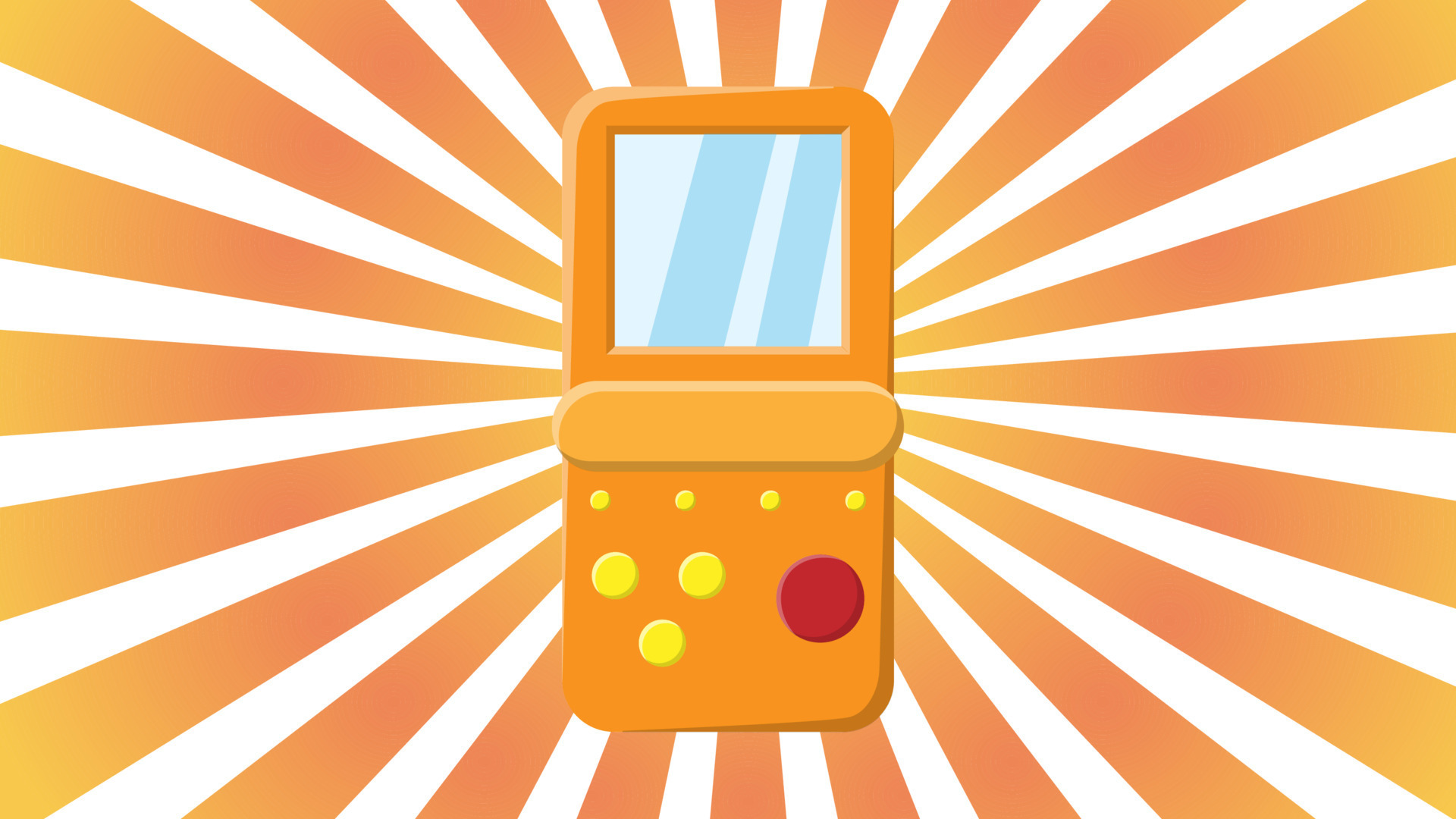This is a detailed cartoon depiction of a retro handheld video game device, primarily colored orange. The device features a square-shaped screen positioned at the top half, with light blue, slanted rectangles indicating light reflection on the front lens. Below the screen, there is a lighter yellow-tan bar across the middle of the device. Arrayed horizontally on the lower left side are four smaller yellow buttons, while a cluster of three slightly larger yellow buttons forms a triangle shape beneath the bar. An even larger red button is positioned to the right of these yellow buttons. The entire device is surrounded by a gradient background of white, dark orange, and light orange rays radiating outward from the device, evoking a visual sense of illumination.